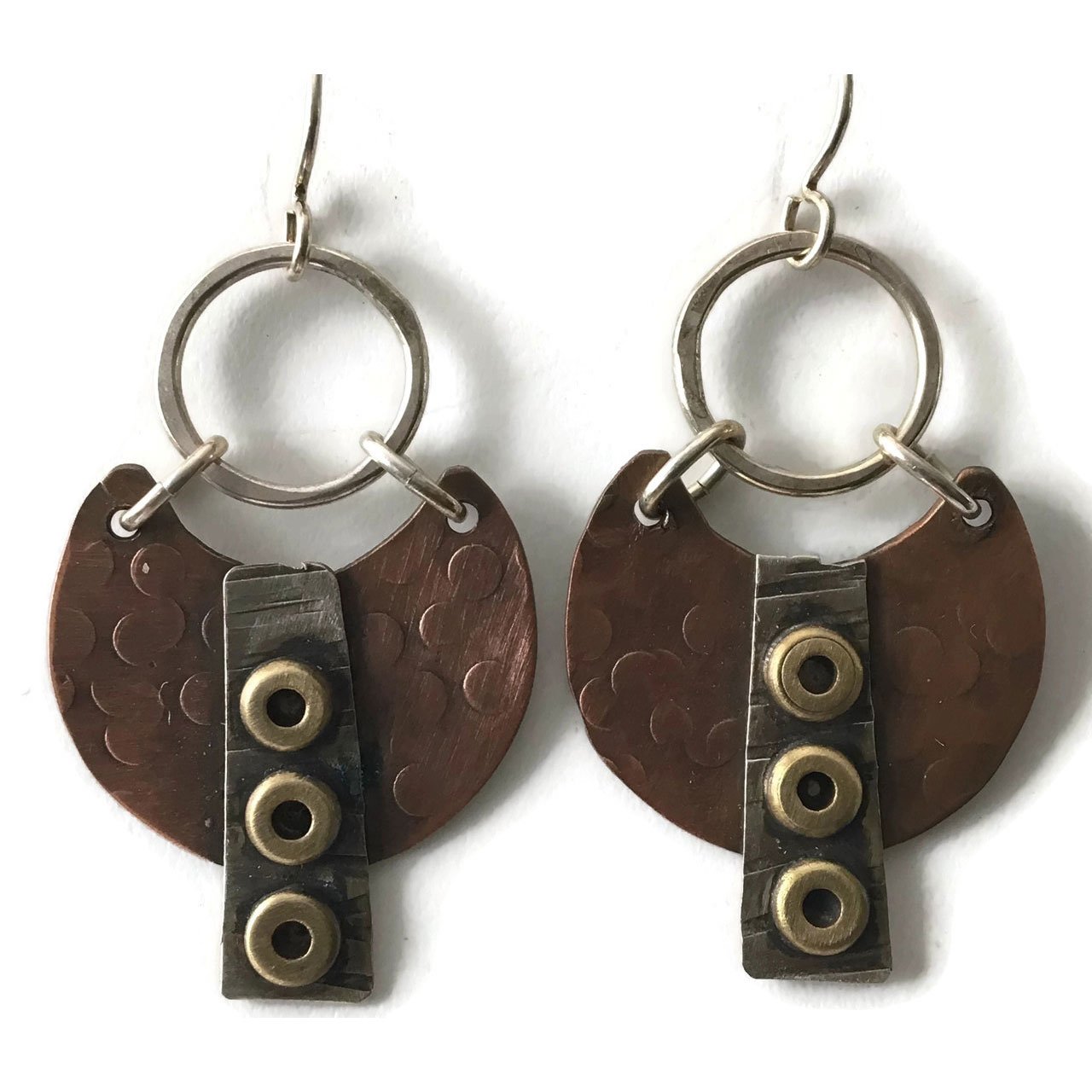This image showcases a unique pair of earrings crafted from silver metal. Each earring consists of a silver hoop with a hook attached at the top, designed for a pierced ear. Dangling from the silver hoop is a moon-shaped, brown disc featuring three golden rings arranged vertically. At the center of the brown disc, there's an additional rectangular brown piece adorned with three bronze-colored holes, adding intricate detail to the overall design. The earrings are artistically fastened with silver connectors, highlighting their distinctive and elegant composition.